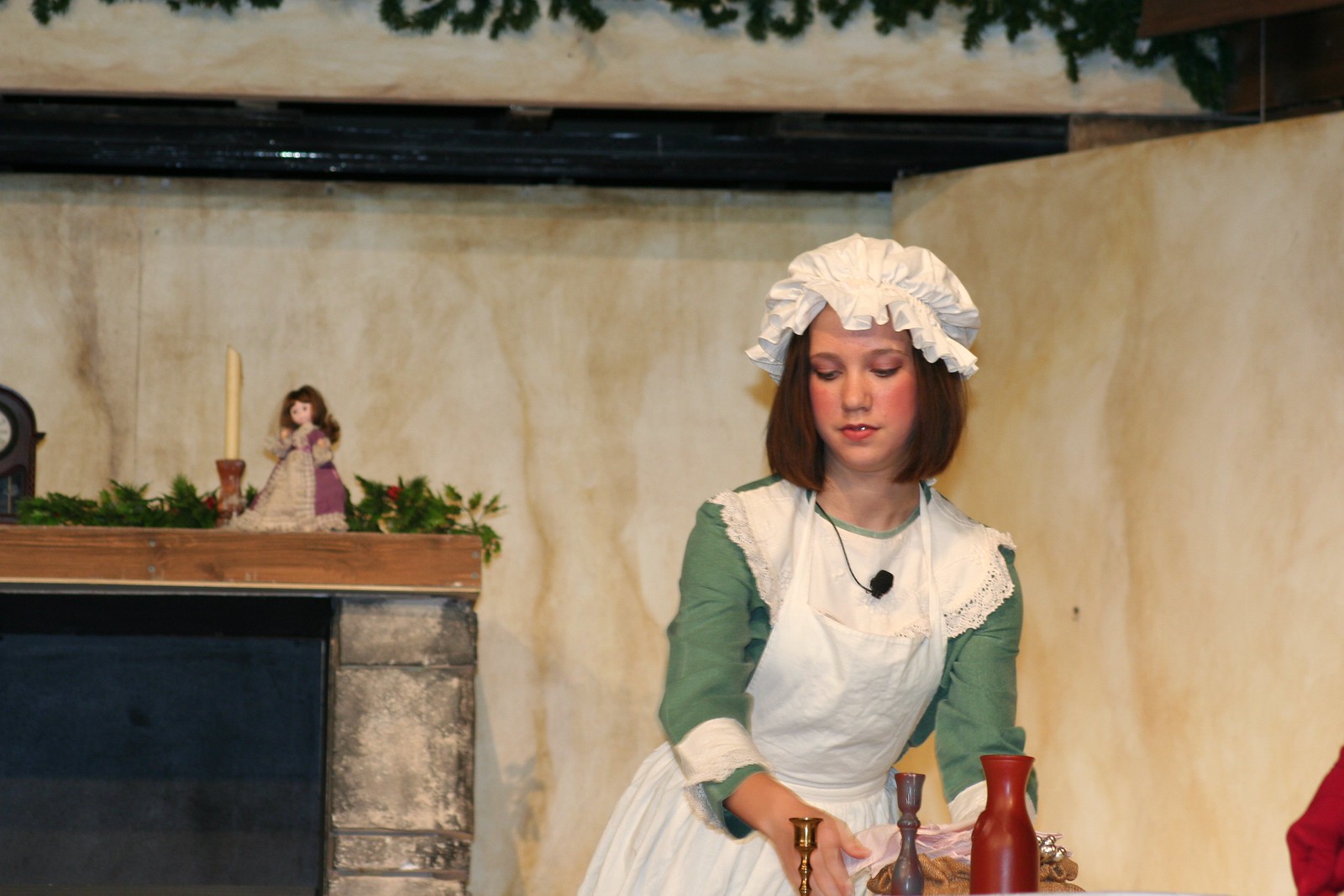This landscape-oriented color photograph captures a young girl, around 15 years old, adorned in a Victorian-era maid's costume. The costume consists of dark green sleeves, a white lacy collar, a white apron, and a white puffy bonnet. She has short to medium-length brown hair and a small microphone attached discreetly to her bonnet, with its wire concealed under her dress.

The girl, slightly right of center and towards the bottom of the frame, is in the midst of arranging items on a table that is not visible. The items include multiple candlesticks, a candelabra, an old-style jug for liquids, and other candle holders. Behind her, a fireplace with a wooden mantel is adorned with an antique-looking doll, a non-burning candle in a candlestick, an old-fashioned clock, and a plastic floral arrangement, which is slightly anachronistic for the colonial or Victorian setting being portrayed.

The overall setting exudes a sense of historical reenactment or stage performance, with the sophistication of photographic representational realism. The background features a beige stucco finish, and some plants hang down across the top, enhancing the period atmosphere.